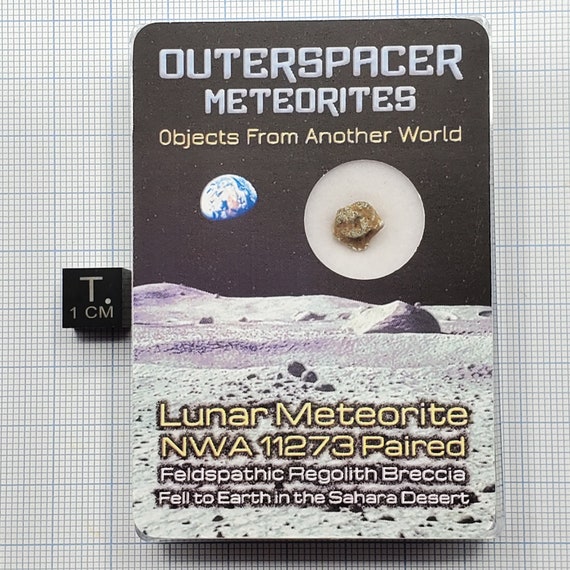This poster features a captivating black background sprinkled with small stars. At the top, large text in white reads "Outer Spacer Meteorites," followed by "Objects from Another World" in striking yellow. Against this cosmic backdrop, a partially obscured photo of Earth is paired with an image of a large, round object that is predominantly white, featuring a brown and gray center. Below, a lunar landscape with white hills and various rocks is depicted. In white text at the bottom, the caption reads: "Lunar Meteorite NWA-11273 paired feldspathic regolith breccia fell to Earth in the Sahara Desert." On the left-hand side of the poster, there's a small black die marked with a gray "T" and "1CM," all positioned on graph paper, providing a scale for the meteorite sample represented.